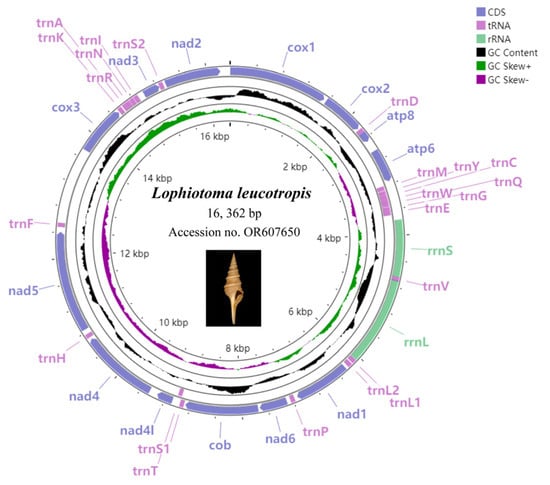This is a detailed scientific diagram depicting the characterization of the mitochondrial genome of *Lophiotoma leucotropis*, a species in the family Turbinellidae, within the Neogastropoda order. The central focus of the diagram is a series of concentric circles representing the genome’s structure. Each circle is subdivided into segments and color-coded corresponding to various genetic components: purple represents CDS, pink indicates tRNA, green signifies tRNA, black denotes GC content, a darker green indicates GC skew, and purple represents GC skew minus.

In the middle of the diagram, the organism's name, *Lophiotoma leucotropis*, is prominently displayed along with the genome size (16,362 BP) and accession number (OR 607650). Below this information, a black rectangle showcases a photograph of the *Lophiotoma leucotropis* snail, characterized by its conical shell with a pointed top and spiral shape.

The outermost circle and some inner circles are segmented and labeled with coded letters and numbers such as CDS, tRNA, rRNA, and other genetic markers like NAD5. Additionally, each segment's respective section is boxed or highlighted in colors corresponding to the genetic components detailed in the legend situated at the top right of the diagram.

Overall, the diagram provides a comprehensive and visually engaging representation of the mitochondrial genetic structure of *Lophiotoma leucotropis*, complete with color-coded annotations and a visual reference to the organism itself, enhancing understanding of this carnivorous snail’s genetic makeup.